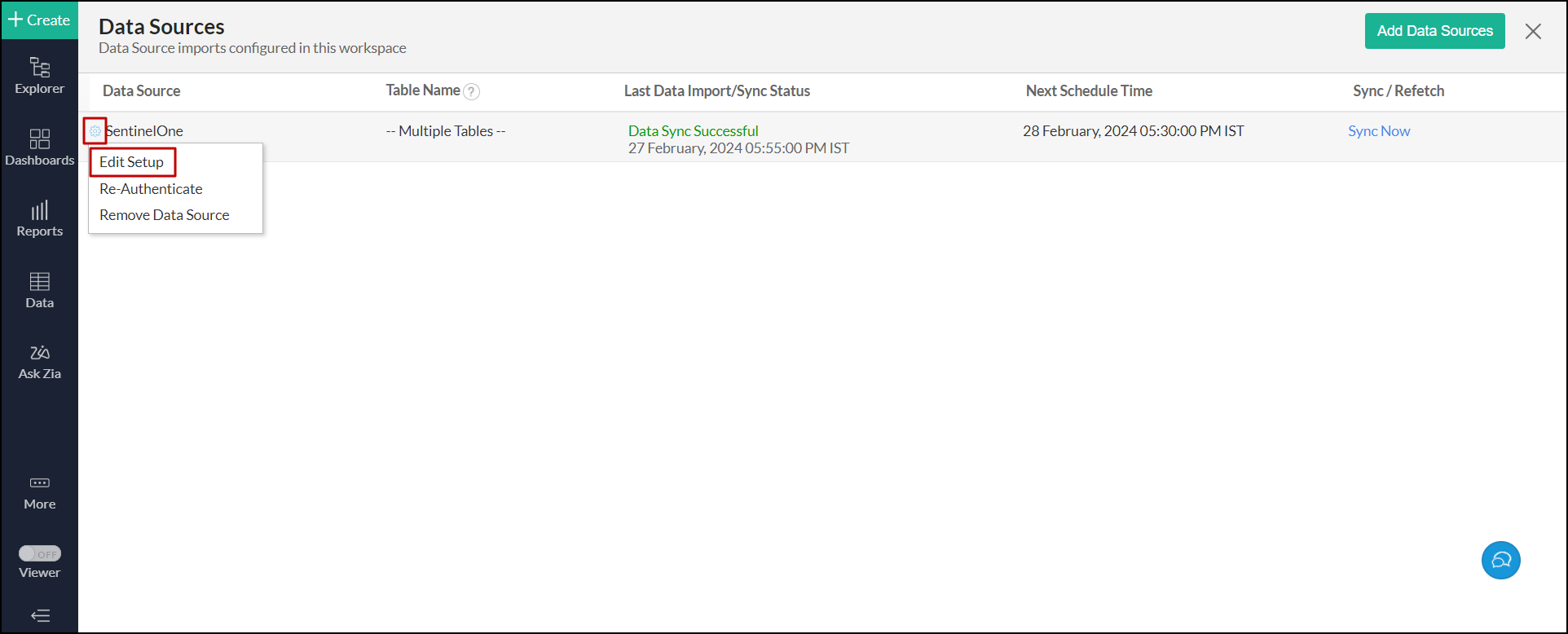In the image, there is a detailed user interface of a data management platform. On the far left side, there's a narrow section featuring the following elements:
- At the top, there's a colored area indicating a tail color.
- Below it, a white plus sign next to the word "Create" over a black background.
- Following this, in white text, there are several options listed vertically: "Explorer," "Dashboard," "Reports," "Data," "Axia," and "More."
- An oval shape in gray containing the text "Off," next to another label "Viewer."
- A graphic with street lines and an arrow pointing left. 

The right section of the interface has a different design and layout:
- It's set against a gray background, with black text labels including "Data Sources," "Data Source Imports," "Data Source," "Table Name," "Last Data Imports," "Last Sync Status," "Next Schedule Time," "Sync," and "Set Refresh."
- Above these labels, there is a green rectangular button with white text that says, "Add Data Sources," and a black "X" icon.

Additionally:
- Below, there is mention of a "Sentinel" data source with an interactive element next to it—a blue gear icon. Clicking this icon appears to open a white pop-up window with black text labeled "Edit Setup," highlighted by a red box.
- Other interactive options in the popup include "RE-AUTHENTICATE" and "REMOVE DATA SOURCE," with each word spelled out individually.
- Within the interface, several notification messages in different colors show the status and time of sync events:
  - In green text, it indicates "Data Sync Successful."
  - Several dates and times are listed in gray text, such as "27 February, 2024, 05:55:00 PM IST," and "28 February, 2024, 05:30:00 PM IST."
  - There's a blue button labeled "Sync Now."

This detailed caption describes all the elements present in a screenshot of a data management system, providing clarity on the functionality and interactive components users can engage with.